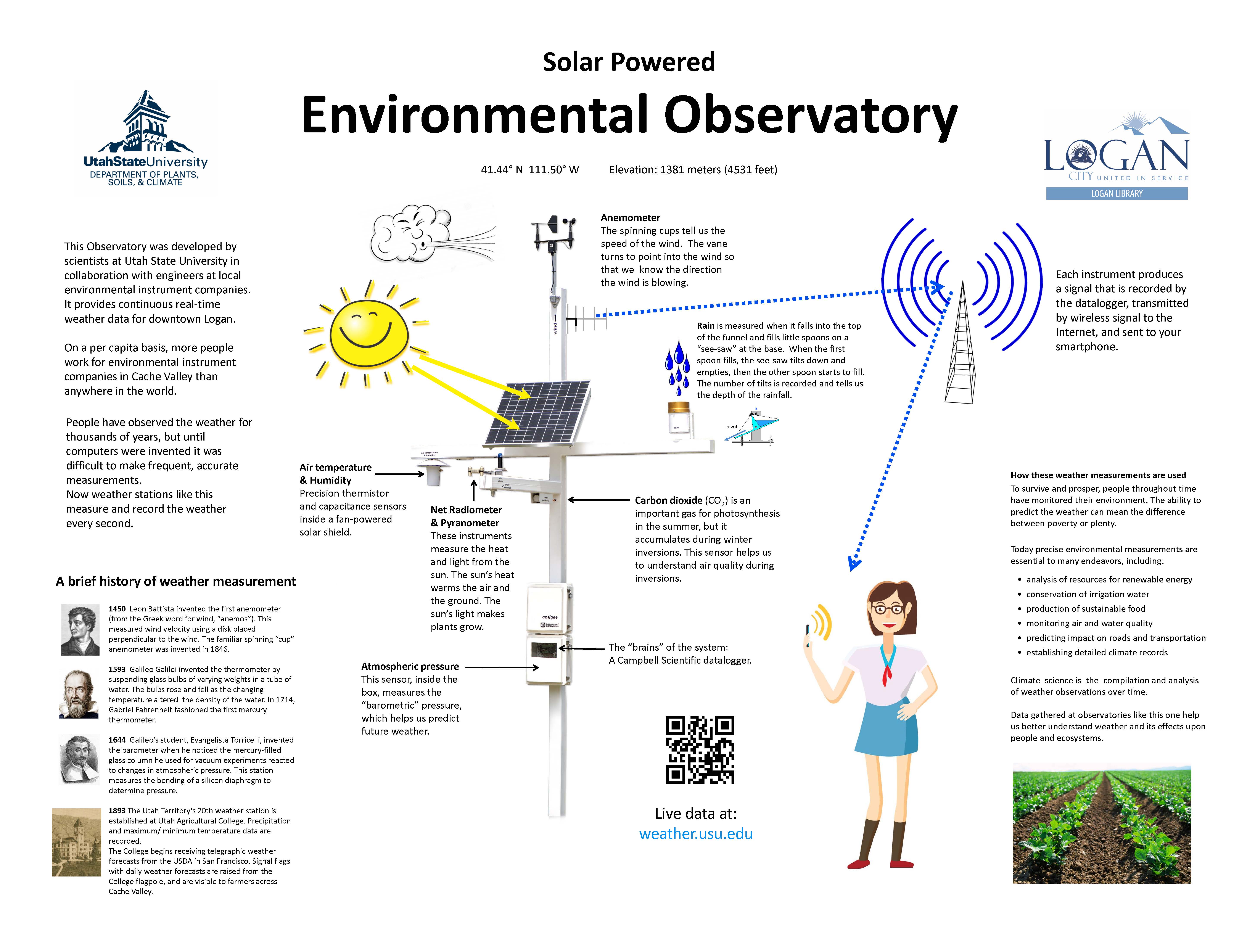The image is an informational chart titled "Cellular Powered Environmental Observatory" displayed prominently in large black text at the top center. Starting from the left, there's a column of black text explaining that this observatory was developed through a collaboration between scientists at Utah State University and engineers from local environmental instrument companies. It provides continuous real-time weather data for downtown Logan. The text goes on to mention that on a per capita basis, more people work for environmental instrument companies in Cache Valley than anywhere in the world. It touches upon the history of weather observation, emphasizing that modern technology now allows for frequent and accurate measurements.

At the center of the diagram are detailed illustrations of the solar panels that power the observatory, with arrows pointing to various components such as the anemometer at the top, which measures wind speed using spinning cups. Below the anemometer is an antenna that wirelessly transmits data to a Campbell scientific data logger, described as the brains of the system. The observatory also includes a solar cell, various sensors for air temperature, humidity, net radiance, power, carbon dioxide, and atmospheric pressure.

Additionally, the bottom of the chart features a QR code that links to live weather data and the bottom right-hand side displays an image of a woman using the weather appliance. The observatory's precise location is marked at 41.44 degrees north and 111.50 degrees west, with an elevation of 1,381 meters (4,531 feet) above sea level. The Utah State University Department of Plants, Soils, and Climate, along with the Logan Library in Logan City, Utah, are credited for this project, showcasing a logo that reads "Logan City United to Service."